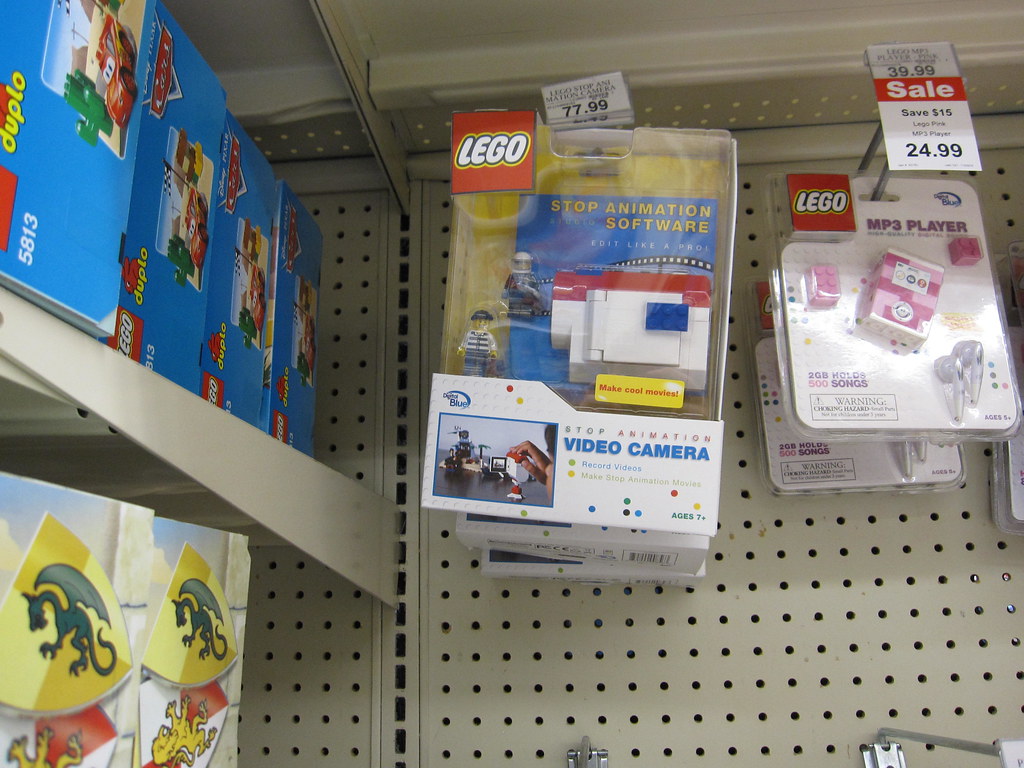This photograph offers a detailed view of a toy store shelf featuring various Lego products. On the far left, there are two metal shelves in light gray or cream color, featuring numerous slots and hooks. At the top of the shelves, there are blue boxes, likely containing Duplo sets, one of which appears to feature a race car. Below these, there are more boxes, including one with what looks like a dragon.

The focal point of the image is a prominently displayed Lego video camera designed for stop animation, priced at $77.99. The packaging shows the red Lego logo in the top left and includes a sticker that touts its capability to create cool movies. To its right, there is a Lego MP3 player, also encased in plastic, with a sale price reduced from $39.99 to $24.99. The MP3 player is red and includes ear plugs, and is capable of storing up to 2 gigabytes or 500 songs.

The photograph captures a typical store display with a close-up perspective, providing a clear view of the assorted Lego products and their prominent positioning on the shelves.